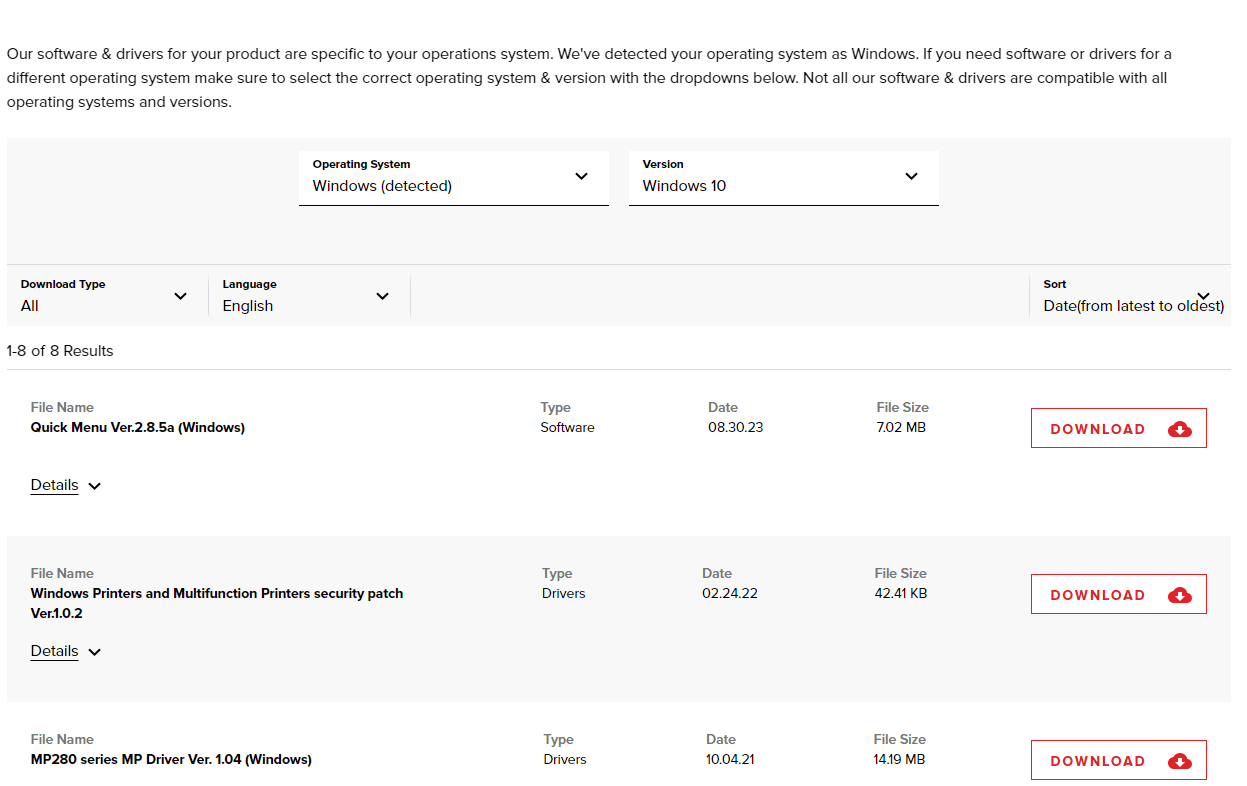The image displays a structured interface for downloading various drivers and patches for the Windows operating system. At the top of the image, there is a notice stating, "Our software and drivers for your product are specific to your operating system. We've detected your operating system as Windows." Users are advised to select the correct operating system and version using the provided dropdown menus if they require software or drivers for a different OS. 

Below this notice, there are two white dropdown boxes with black text. The first box on the left shows "Operating System: Windows (detected)" with a dropdown arrow for adjusting the OS. The second box, positioned slightly to the right, specifies "Version: Windows 10" with another dropdown arrow.

Further down, there is an additional section allowing users to refine their search by selecting "Download Type" (defaulted to "All"), "Language" (defaulted to "English"), and sorting options by "Date: Latest to Oldest." The section indicates displaying "1 to 8 of 8 results."

The results section consists of columns for File Name, Type, Date, and File Size:
1. "Quick Menu version 2.85 (Windows)" listed as Software, dated "8-30-23," with a file size of "7.02 MB." Details can be expanded.
2. "Windows Printers and Multifunction Printer Security Patch version 1.02" listed as Drivers, dated "02-24-22," with a file size of "4241 KB." Details can be expanded.
3. "MP280 series MP Driver version 1.04 (Windows)" listed as Drivers, dated "10-04-21," with a file size of "14.19 MB." Details can be expanded.

Each file listing includes a download button, which is a white rectangle with a red border and the word "Download" in red text. Next to this is a download icon, represented by a cloud with a downward-pointing arrow.